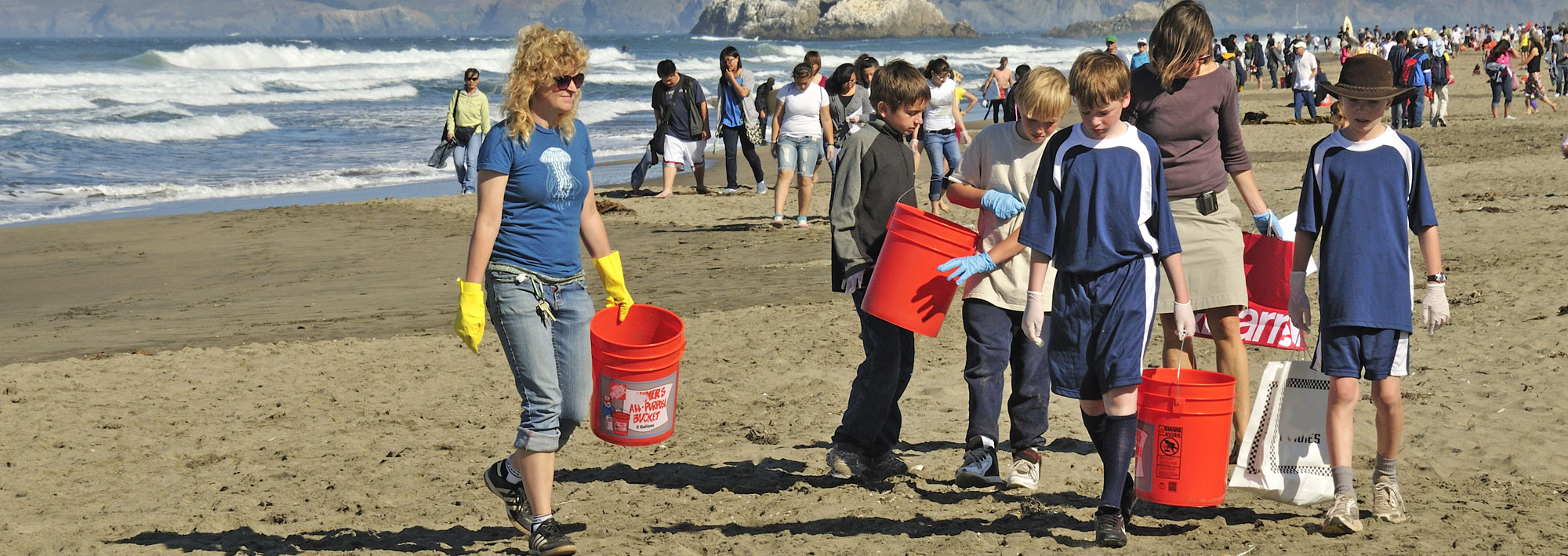This is a detailed photo of a beach cleanup scene in a landscape view, depicting a vibrant community effort. In the foreground, a group of children and two women are prominently featured. The woman in the front and center is wearing a blue t-shirt and blue jeans rolled up to her knees. She is accessorized with yellow gloves, sunglasses, long blonde hair, and has keys hanging from a belt loop. She carries an orange bucket with determination. Surrounding her are children also involved in the cleanup, each holding orange buckets and wearing a mix of white and latex gloves. In the background, large crowds of people can be seen near the water, busy with their own cleaning tasks. The beach sand is a light brown color, and to the left, the ocean waves crash actively onto the shore, creating a dynamic white froth against the light blue sea. The overall scene captures the collective effort and dedication of the community to keep the beach pristine.